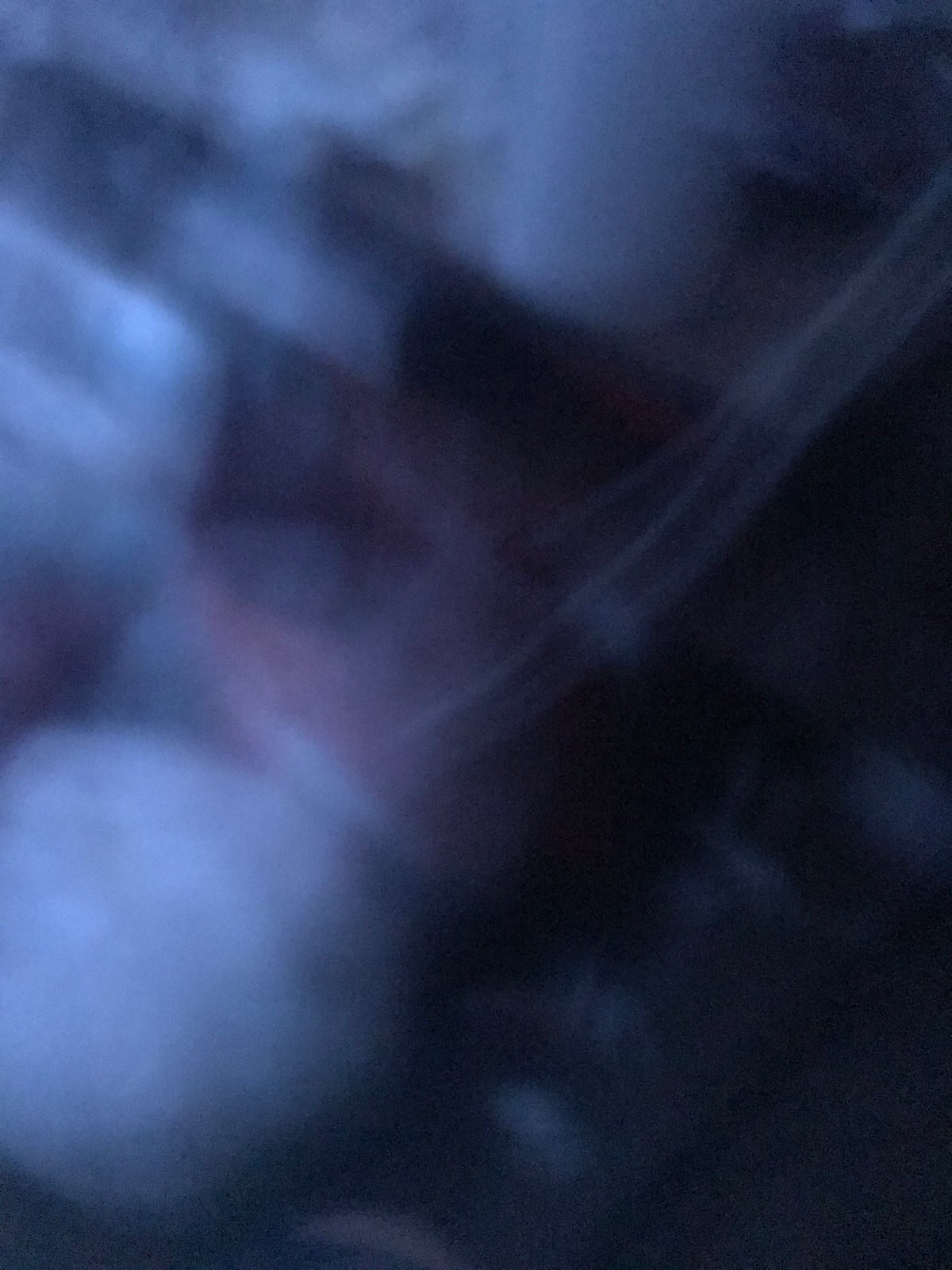The image presents a visually striking composition with a combination of colors and shades. In the top left corner, a pristine white segment gradually transitions into a light blue hue. This light blue shade also makes an appearance in the bottom left corner. Dominating the center of the image is a stark black area, which extends towards the bottom right, creating a bold contrast. The bottom right is particularly dark, with dense black tones, while the right side of the image also features considerable black coverage. Adding to the dynamic range of the image, the top left and bottom left corners are infused with shades of light blue, counterbalancing the presence of black. The center of the image displays a striking patch of white, breaking the continuity of darker shades, making the composition both captivating and complex.